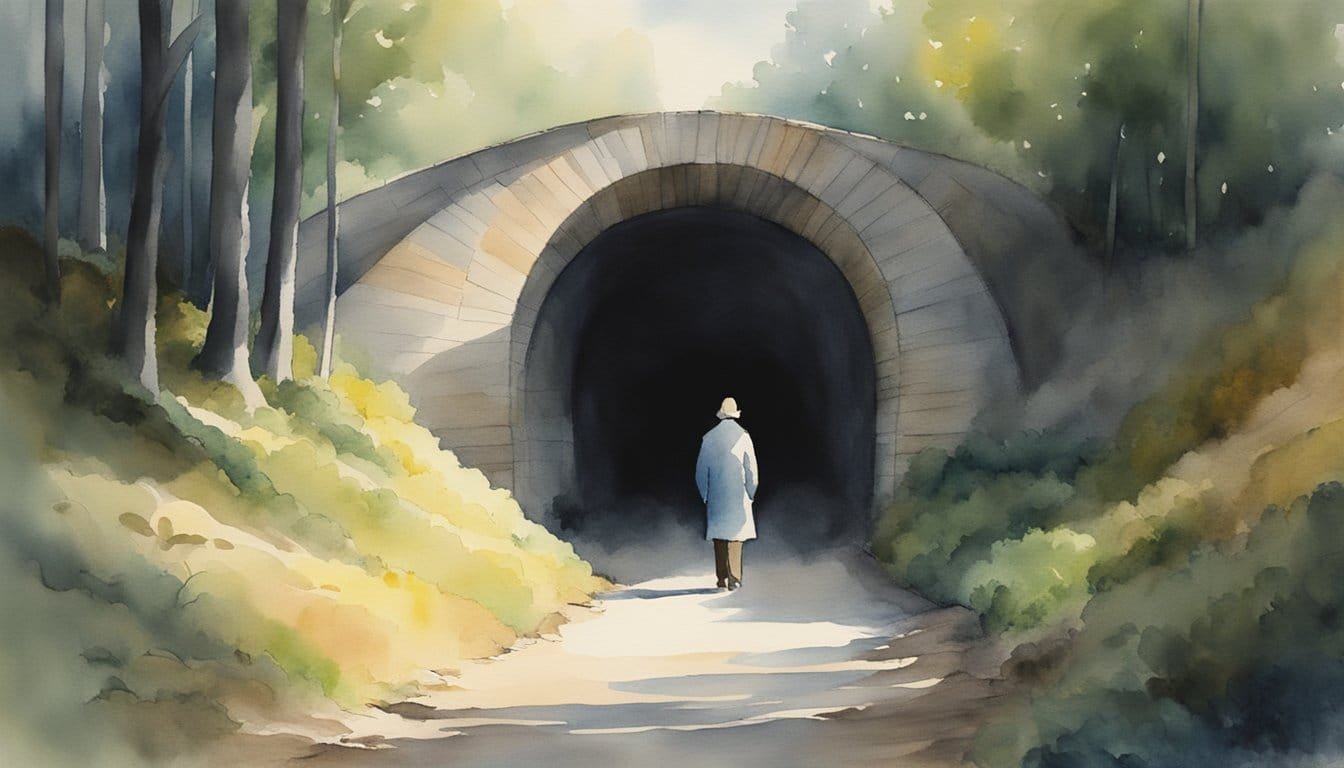This image is a serene and peaceful depiction of a man walking towards a dark tunnel in an outdoor, daylight setting. Rendered in a simplistic watercolor style with little to no outlines, the artwork captures a natural scene dominated by hues of yellow, green, and gray. The man, positioned centrally, wears brown pants, a blue trench coat, and a yellow hat. He is walking along a dirt pathway that leads into a tunnel characterized by a large stone archway made of red, light blue, and yellow bricks. Surrounding the path and tunnel are gently sloping hills adorned with a mixture of light and dark green bushes, grasses, and tall trees climbing up both sides. Above and behind the tunnel, the sun filters through additional green trees, creating a peaceful and serene atmosphere that shows the tunnel nestled in the heart of nature.